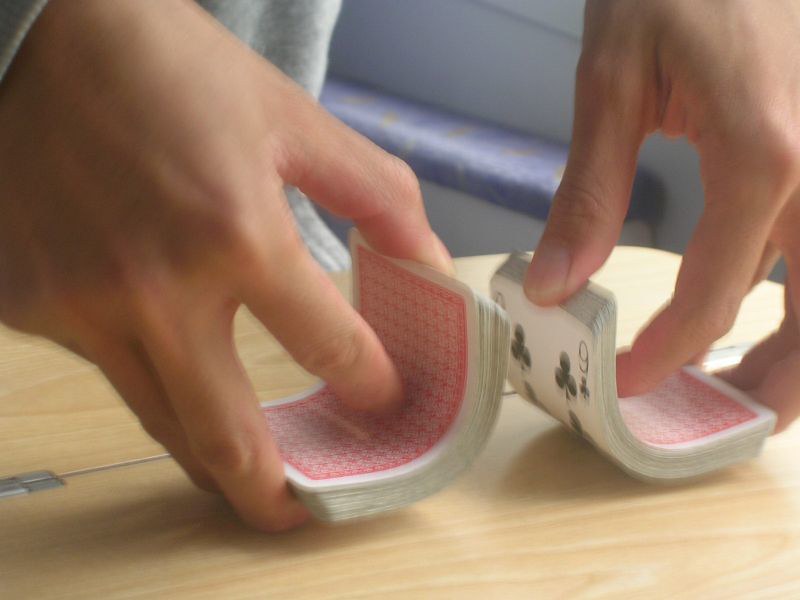In this slightly blurry photograph, a pair of Caucasian male hands are caught mid-motion as they skillfully shuffle a deck of cards on a light wooden table. The hands, gripping the cards with a practiced hold, are positioned in such a way that the deck has been split in half, each half lying face down on the table. The table itself features a distinct silver hinge, indicating it is a foldable piece of furniture. Among the cards, one stands out with its face clearly visible—the nine of clubs, its black suit starkly contrasting against the shuffled deck. The remaining cards reveal their red and white patterned backs, adding a hint of vibrancy to the scene. The man is dressed in a gray sweatshirt, a sleeve of which drapes slightly over the wrist of his left hand. The background of the photo is a soft blue, providing a calming backdrop to the dynamic action of the card shuffle.